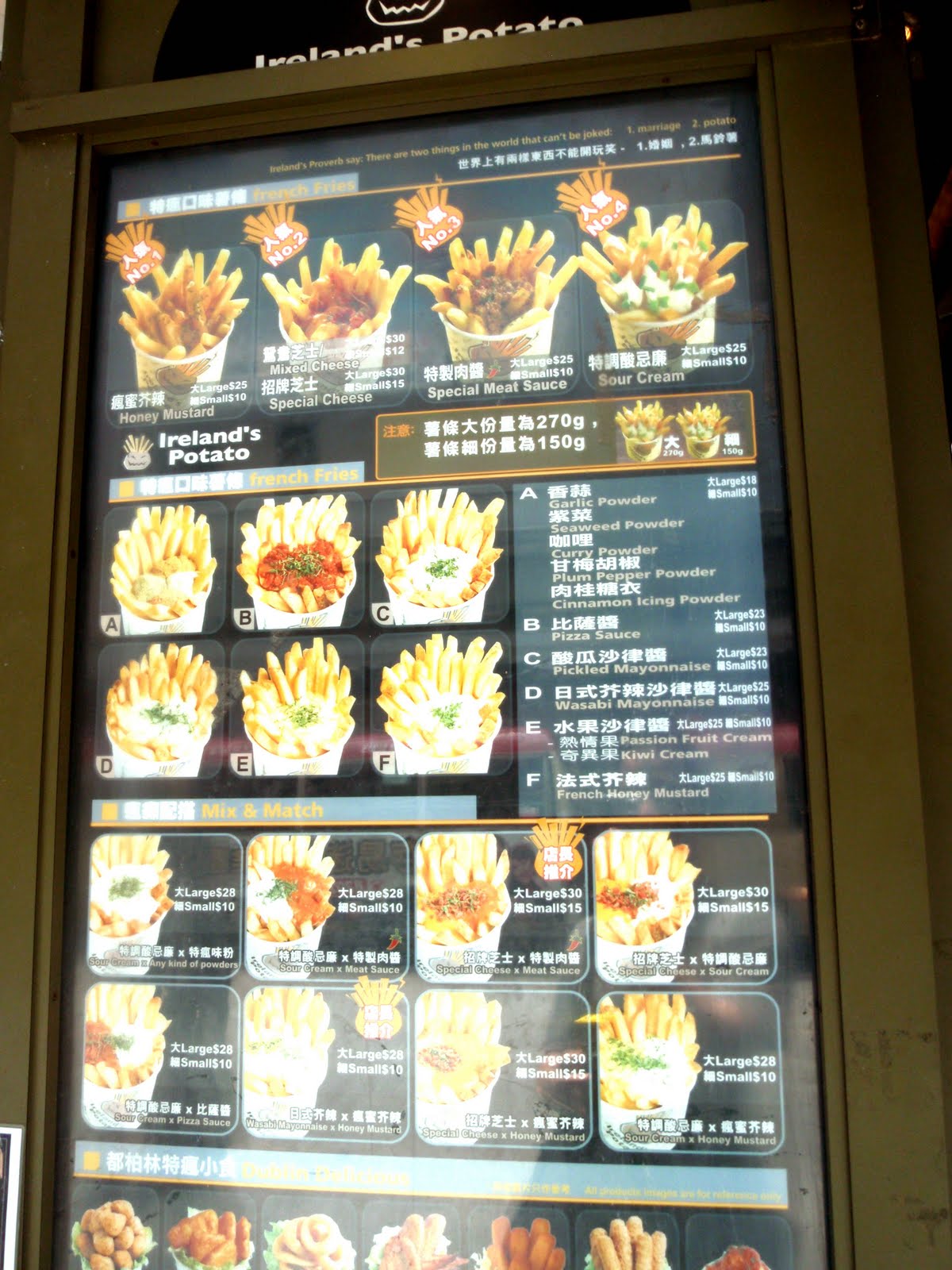The menu board inside this restaurant, possibly named "Ireland's Potato," features an array of dishes centered around French fries, written predominantly in Japanese. The offerings all involve creative variations of French fries or potato-based products. Some items appear to be simple servings of French fries in cups, topped generously with a variety of sauces or fillings, such as chili, ketchup, ranch dressing, or other delicious toppings. While the precise names of the dishes are not discernible due to the Japanese text, the English phrase "Ireland's Potato" stands out, possibly indicating the theme or name of the establishment. The menu presents a visually appealing assortment of French fry creations, each promising a unique and flavorful experience.